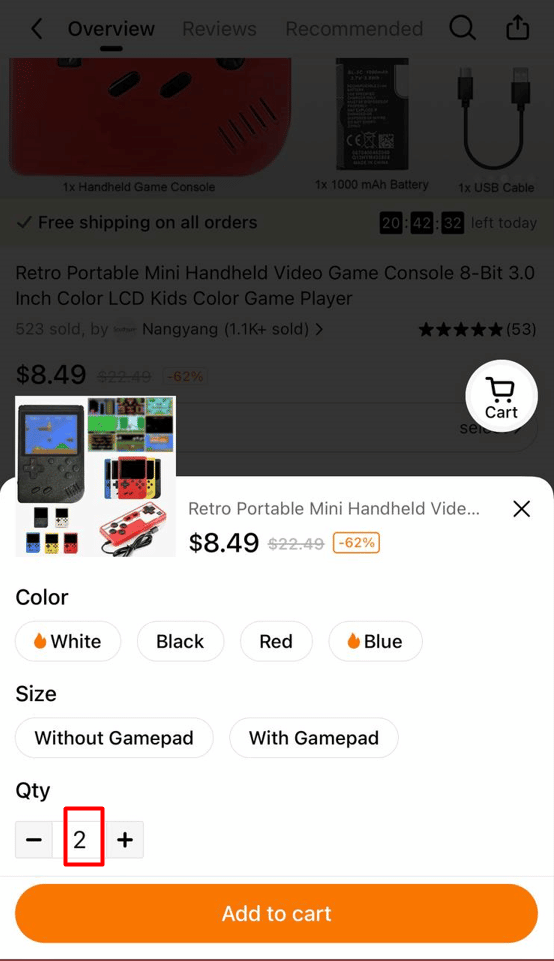A detailed screenshot is captured from a mobile device displaying a shopping website. The top part of the screen is obscured due to an overlay or a pop-up relating to the item being viewed. The focus of the screen is on a retro portable mini handheld video game console reminiscent of a Gameboy but seemingly a third-party knockoff version. It is labeled as an 8-bit video game console featuring a 3.0-inch color LCD. The console is designed primarily for kids and offers a colorful gaming experience.

Several color options are available for the device, including white, black, red, and blue. Notably, there is an option to purchase the console either with or without an additional gamepad, which serves as a detachable controller enhancing the gaming experience. The quantity selected for purchase is two, highlighted by a red square around the number two. Positioned at the bottom of the screen is an orange "Add to Cart" button, inviting the user to finalize their selection.

The item is currently on sale, with a significant discount reducing the original price from $22.49 to $8.49.